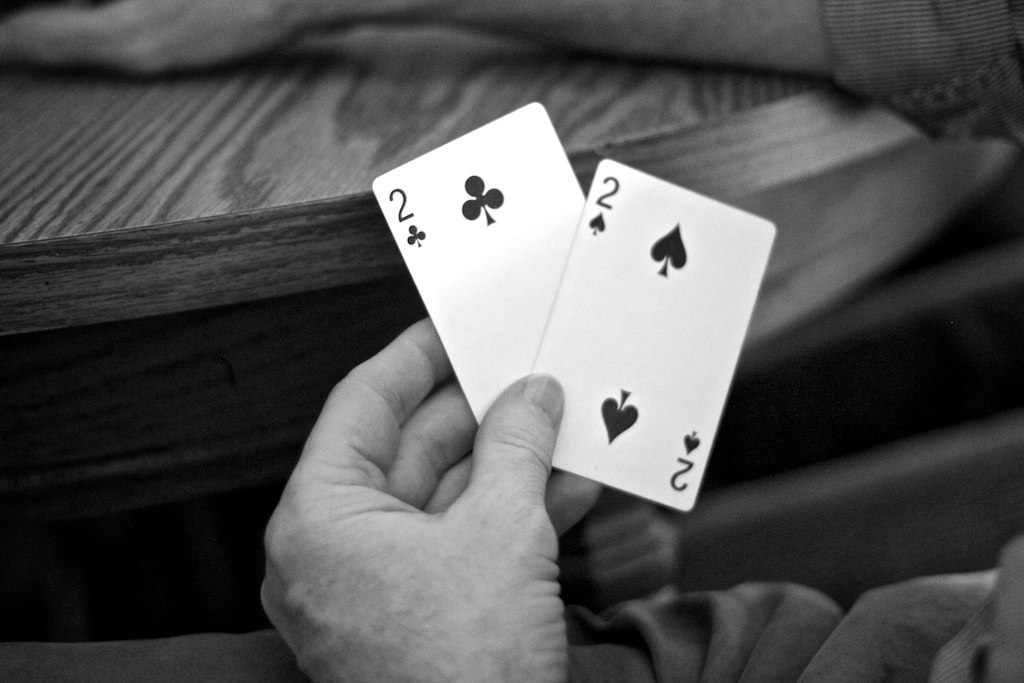In this black and white photograph, a man presumably in his fifties is depicted holding two playing cards in a close-up shot. The scene is set around a small, circular wooden table. The man, likely of Caucasian descent, is seated with his left hand resting on his leg and his right arm positioned on the table's surface.

The image captures just the bottom of his pant leg, his left hand, part of the table's side, and a portion of the table top showing the man's thumb, forearm, and a bit of his ribbed, corduroy-like sleeve. The cards he holds in his left hand are the two of clubs and the two of spades, displayed in a V-shape with the two of clubs slightly higher and angled towards the top left corner. The photograph's subtle textures and the muted black and white palette add a timeless, nostalgic quality to the scene.